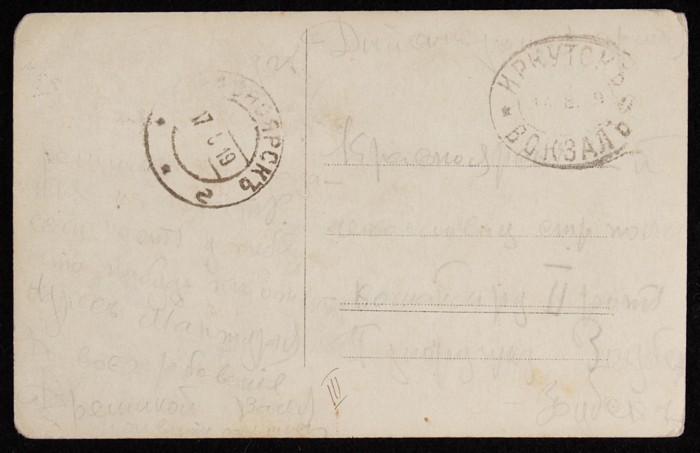This image features the back of a very old and faded tan postcard. The postcard appears to be mounted on a black border or it might be part of the design. Both its age and condition are evident from its yellowed, dirty appearance and opaque, smeared pencil marks. The writing, which is not in English, is faint and slanted, making it almost illegible. At the top right corner of the postcard, there are two postage stamps, one prominently featuring the numbers 14, 8, and 9 and written in what appears to be Russian. The left side also bears a circular stamp with the numbers 17, 6, and 19, again possibly in Russian. The right-hand side of the postcard is lined, suggesting this area was meant for the address, while the left side contains a faded message. An additional notable detail is the presence of a Roman numeral III at the bottom right of the card. The overall impression is one of an antiquated and worn correspondence item with many details lost to time.